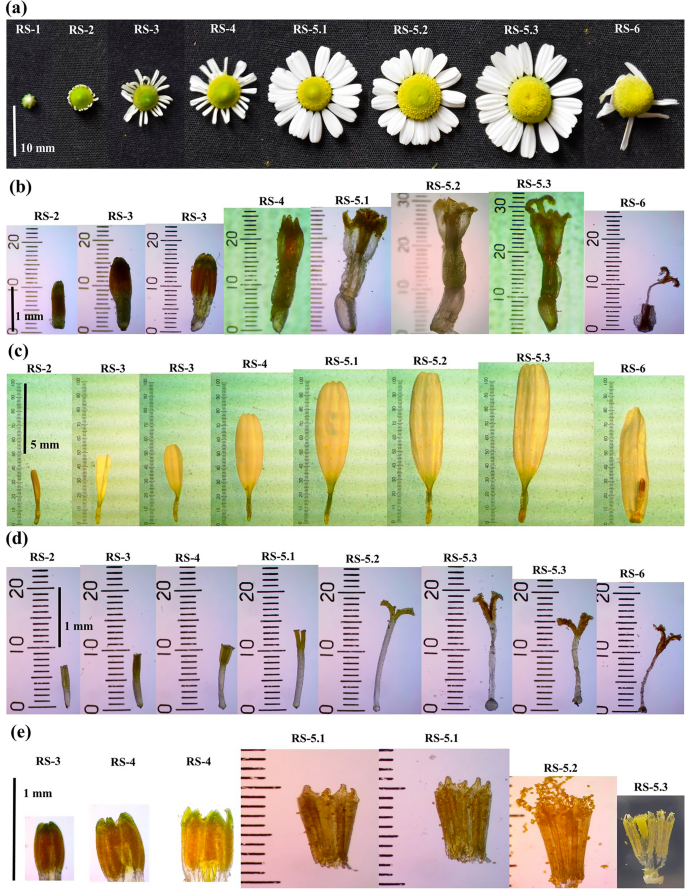This scientific photograph showcases the developmental stages of various flowers arranged meticulously in five rows against a black background. Each row documents the progression from the initial growth phase to full maturity and eventual decay.

- **First Row**: Displays flowers transitioning from tiny buds to mature, blooming flowers. These flowers predominantly exhibit green and white hues.
- **Second Row**: Features images marked with blue and purple calibrations, detailing the height measurements of the flowers as they grow.
- **Third Row**: Similar to the second row, it includes green calibrations for height measurement, highlighting the lifecycle of yellow flowers. These flowers are shown growing, flourishing, and then gradually withering.
- **Fourth Row**: Contains bluish-purple markings to track the height of the flowers, capturing their entire lifespan from blooming to decay.
- **Fifth Row**: Presents flowers with accompanying codes for identification, illustrating their growth stages—from initial white stems to green buds and eventual withering.

Throughout the image, the transition of the flowers is meticulously detailed, highlighting their progression from budding to full bloom and ultimately to their decline, illustrating the cyclical nature of plant life.